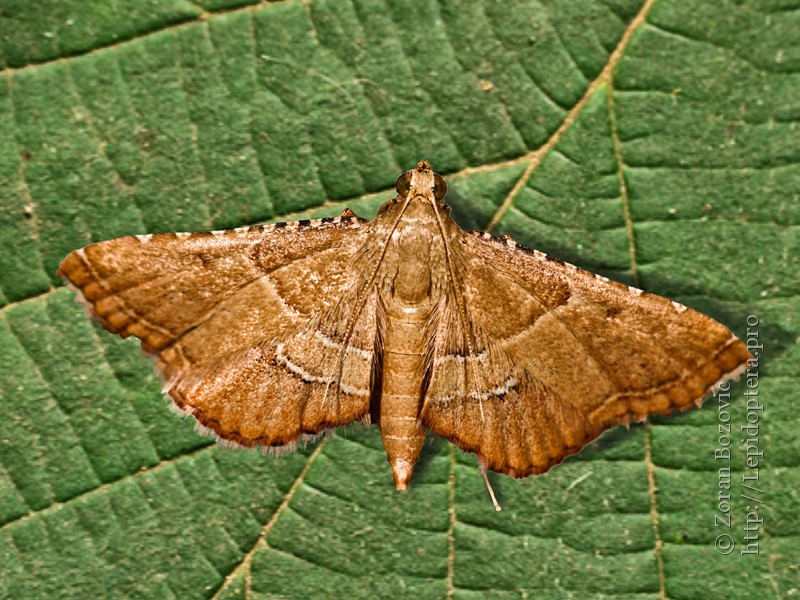A highly detailed nature photograph captures a close-up of a textured green leaf with distinctive tan veining. Centered on the leaf is a light brown moth, shown with remarkable clarity. The moth's forewings display a mix of dark brown and white patterns along their margins, including wavy lines closer to its body and fine, hair-like projections along its hindwings. Notably, the moth's antennae are laid back, resting along its back. Its medium brown eyes and intricate wing details, including white triangles and lines, are clearly visible. The green leaf fills the entire background of the image, providing a vivid contrast to the moth's earthy tones. A watermark vertically aligned on the right-hand side reads "copyright Zoran Bozovic, http://lepidoptera.pro," indicating the photographer specializes in lepidopterans—moths and butterflies.